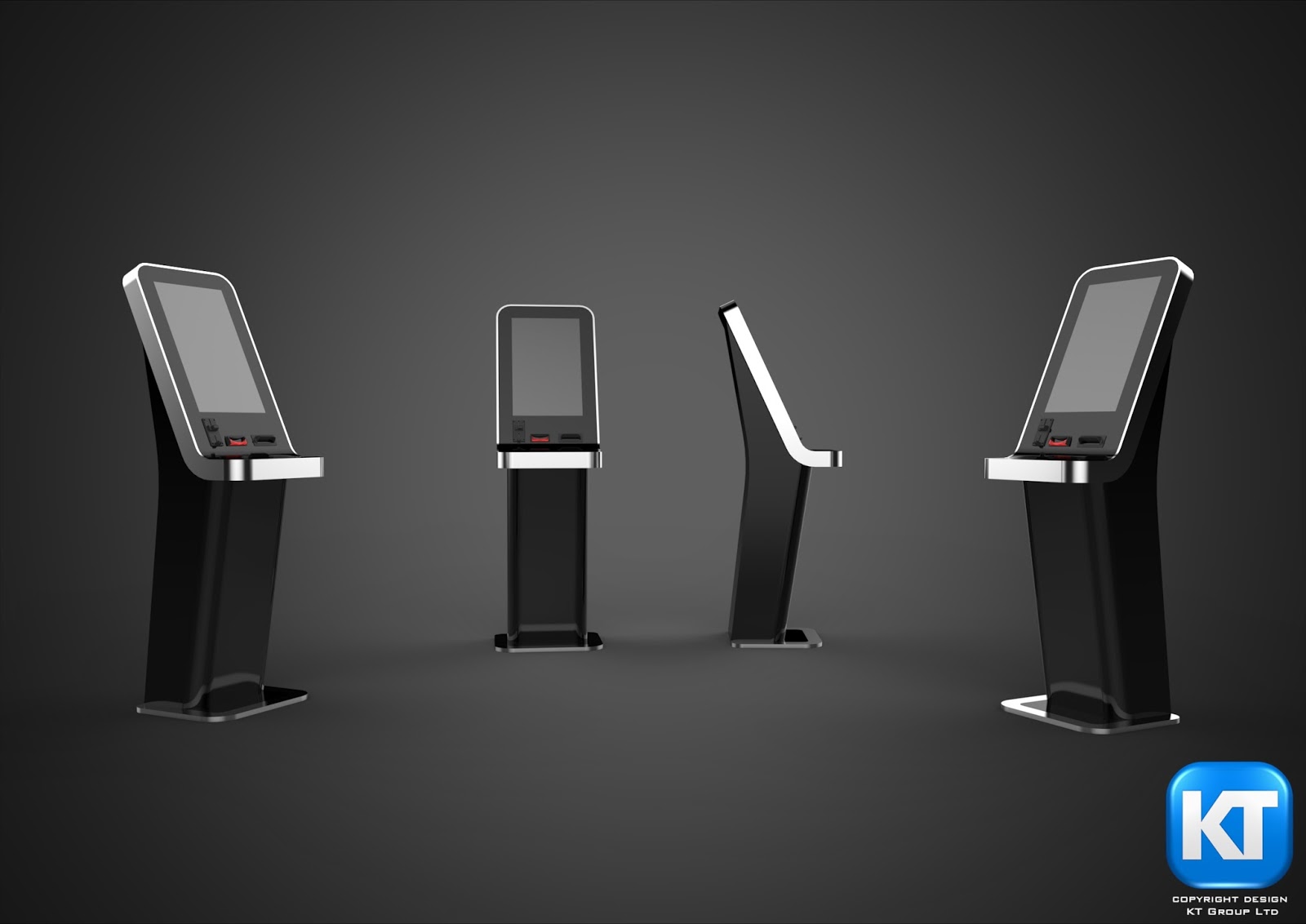This detailed 3D color illustration in landscape orientation depicts four views of a pedestal monitor, reminiscent of kiosks or charging stations. The monitors have a black rectangular base, slightly pitched forward, supporting a vertically oriented screen with a chrome surround and a projecting shelf at the front, accompanied by control buttons. The four views include a left-facing angle, a straight-on front view, a side profile, and a right-facing angle, all suggesting independent, ATM-like kiosks with variable perceived sizes. The background is a dark gray gradient that lightens toward the center. In the lower right corner, there is a blue square with white text reading "KT" and a small note below stating "© design by KT Group Limited." The overall aesthetic suggests a sleek, futuristic design with attention to detail and user interaction.